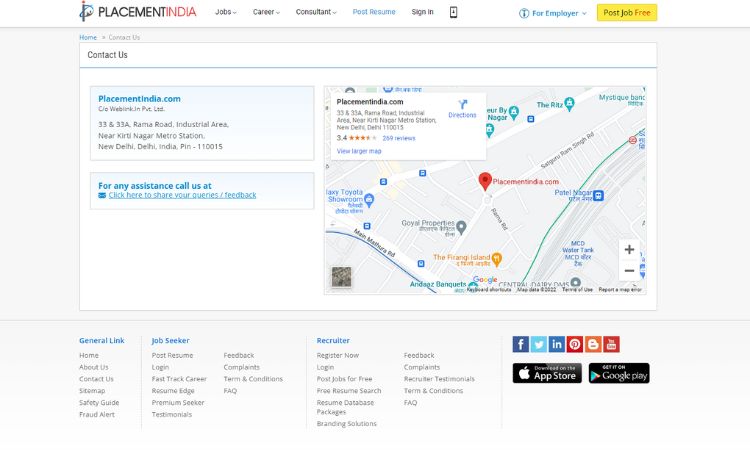In the predominantly off-white or light gray image, the top section features a white banner bar with various elements. Starting from the left, there is a logo that resembles a fish head with a baton passing through it, though this might be a misinterpretation. This is followed by the words "PLACEMENTINDIA" in all caps, where "PLACEMENT" is in black and "INDIA" is in red. 

To the right of this, there are menu options: "Jobs," "Career," and "Consultant," each in black font with small initial letters and a drop-down menu indicated beside them. Following these options, "Post Resume" is written in blue font, then "Sign-In" in black, and a black cell phone icon. Next, there is a blue icon resembling an eye, potentially indicating information, accompanied by "For Employer" in blue font with a drop-down menu.

Further to the right, there’s a prominent yellow button that reads "Post Job Free," with "Post Job" in black and "Free" in red. Below the banner, there is a smaller navigation option with "Home" in blue and "Contact Us" in gray.